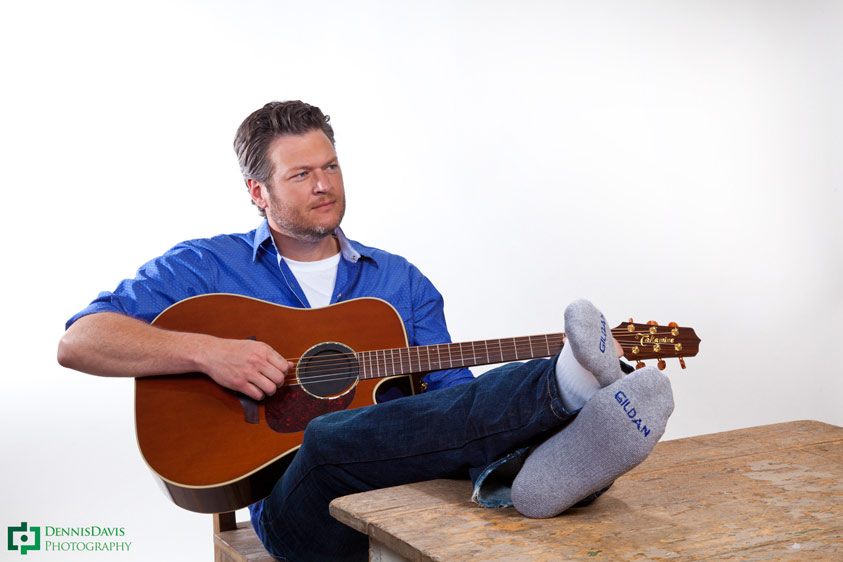In this photograph, a man, identified as Blake Shelton, is seated on a chair with his legs crossed atop an old, heavily worn wooden table. The table, distressed with much of its varnish gone, serves as a resting place for his socked feet. His gray-and-white sock soles display the brand name 'Gildan' in blue letters. Dressed casually, he wears dark blue jeans paired with a light blue button-up shirt, the sleeves rolled up past his elbows with the top four buttons undone, revealing a white crew neck undershirt. The man cradles a dark brown acoustic guitar with white trim, focusing on its strings as he looks off to something on the right, possibly singing. The backdrop is a plain white, and in the bottom left corner, the image is credited to Dennis Davis Photography in green text.